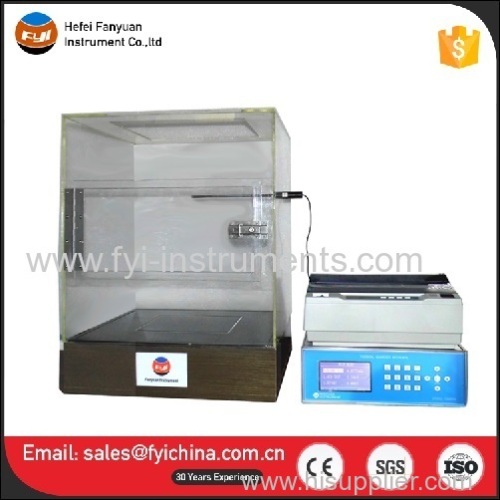This promotional image for an electronic device features a detailed scientific instrument prominently displayed against a white background with a black border. The central focus is a large transparent box on the left, sitting on a wooden base, equipped with a door latch and connected by a black wire to a smaller beige electrical machine on the right. The smaller instrument has a beige upper part with a black top, featuring small white buttons, and a blue lower part displaying an LED screen.

In the top left corner of the image, there is a blue, orange, and black globe-like logo with white text reading "FYI." Adjacent to this, in black text, is the company name "F.A. Fenyon Instrument Co. Ltd." On the top right corner, there's a gold emblem resembling a dollar symbol.

At the bottom, a red banner provides an email address: sales@fyi-china.com.cn. Below this, a black bar highlights "30 years experience" and includes three certification logos: CE, SGS, and ISO. Additionally, a faint watermark at the bottom reads www.hissupplier.com. Textual elements like the website URL www.fyi-instruments.com also appear at the top, enhancing the promotional message.